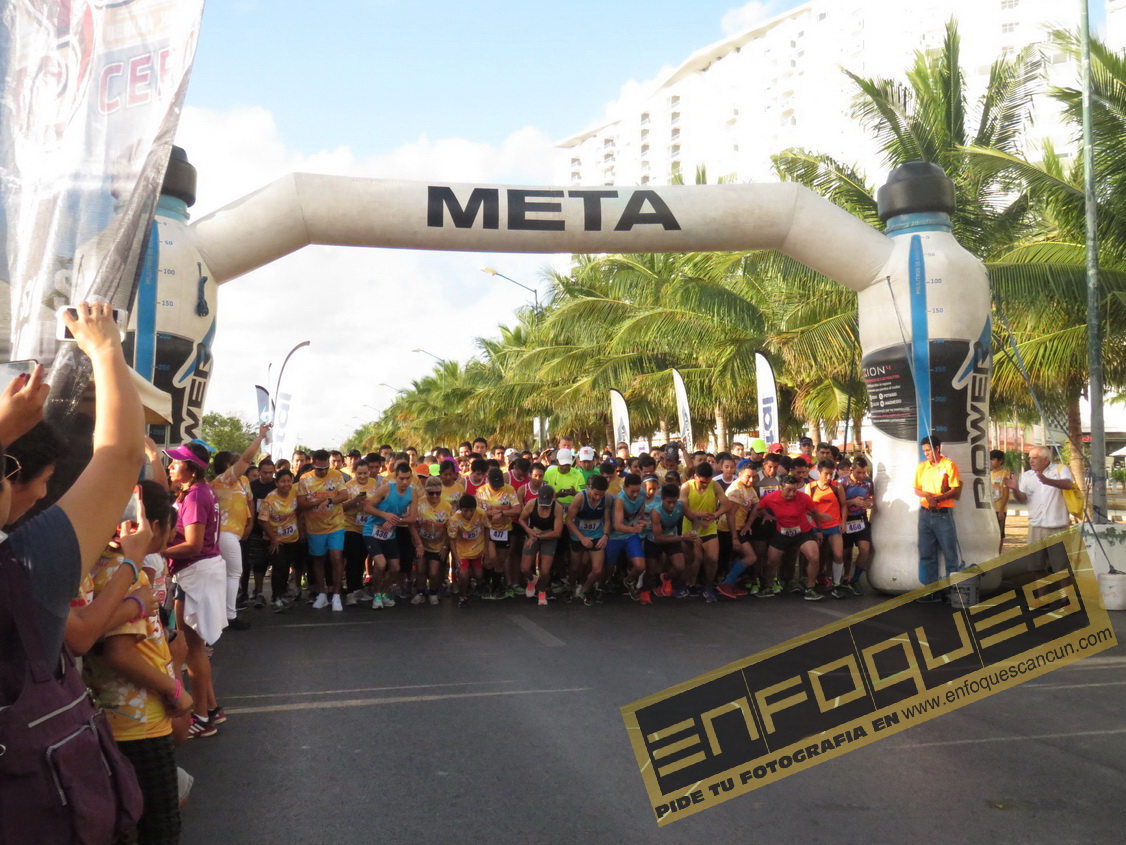This vibrant, full-color photograph captures a lively outdoor scene during the daytime in Cancun, as indicated by the palm trees lining the street and the website InfocaseCancun.com present at the bottom of the image. The focal point is a crowd of participants poised at the starting line of a race, gathered under a large inflatable arch adorned with sponsor names META in bold black text and Powerade. The sky is clear and blue, enhancing the tropical ambiance. Tall buildings, possibly hotels, stand in the background, adding to the urban atmosphere. Onlookers line the sides of the road, cheering on the racers who are dressed in various brightly colored shirts. The cement pavement stretches ahead, marking the path the participants will soon race upon.